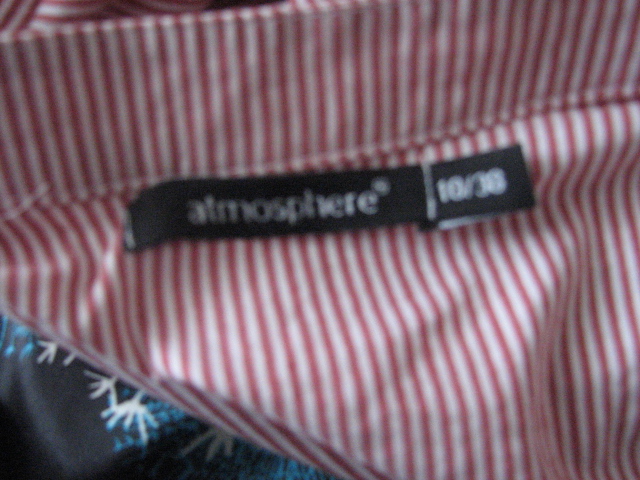This image features a close-up of an article of clothing that is predominantly white with vertical red stripes. The fabric appears to be part of a shirt. At the top of the garment, there is a black label with white lettering that reads "ATMOSPHERE," and beside it, a smaller black tag indicates the size as "10/38." In the bottom left corner of the photo, there is a separate piece of dark blue fabric, almost black in color, adorned with white patterns resembling small branches or snowflakes, and light blue dots scattered throughout. The image itself is quite blurry, making the finer details hard to discern.